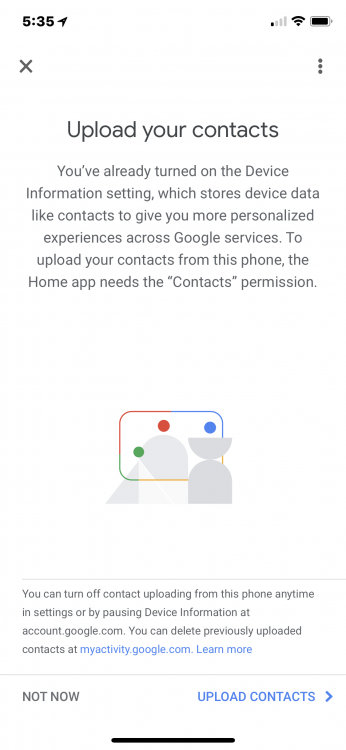Screenshot of a smartphone displaying a Google service prompt. The screen captures a request to upload contacts, explaining that the user has already activated the device information setting, which stores device data such as contacts to provide personalized experiences across Google services. Emphasized text informs that the Google Home app requires contact permission to upload contacts. 

A colorful icon, with a rounded rectangle featuring a green dot, red dot, blue dot, and various geometric shapes, is situated prominently in the interface. The prompt reassures that contact uploading can be disabled at any time via settings or by pausing device information at account.google.com. It also offers instructions for deleting previously uploaded contacts at myactivity.google.com and includes a "Learn More" link for additional information.

At the bottom, the user is presented with two options: "Not now" or "Upload contacts." The top status bar shows it is 5:35 PM, with the phone connected to a full Wi-Fi signal but only one bar of cellular signal reception. The battery icon indicates a full charge.